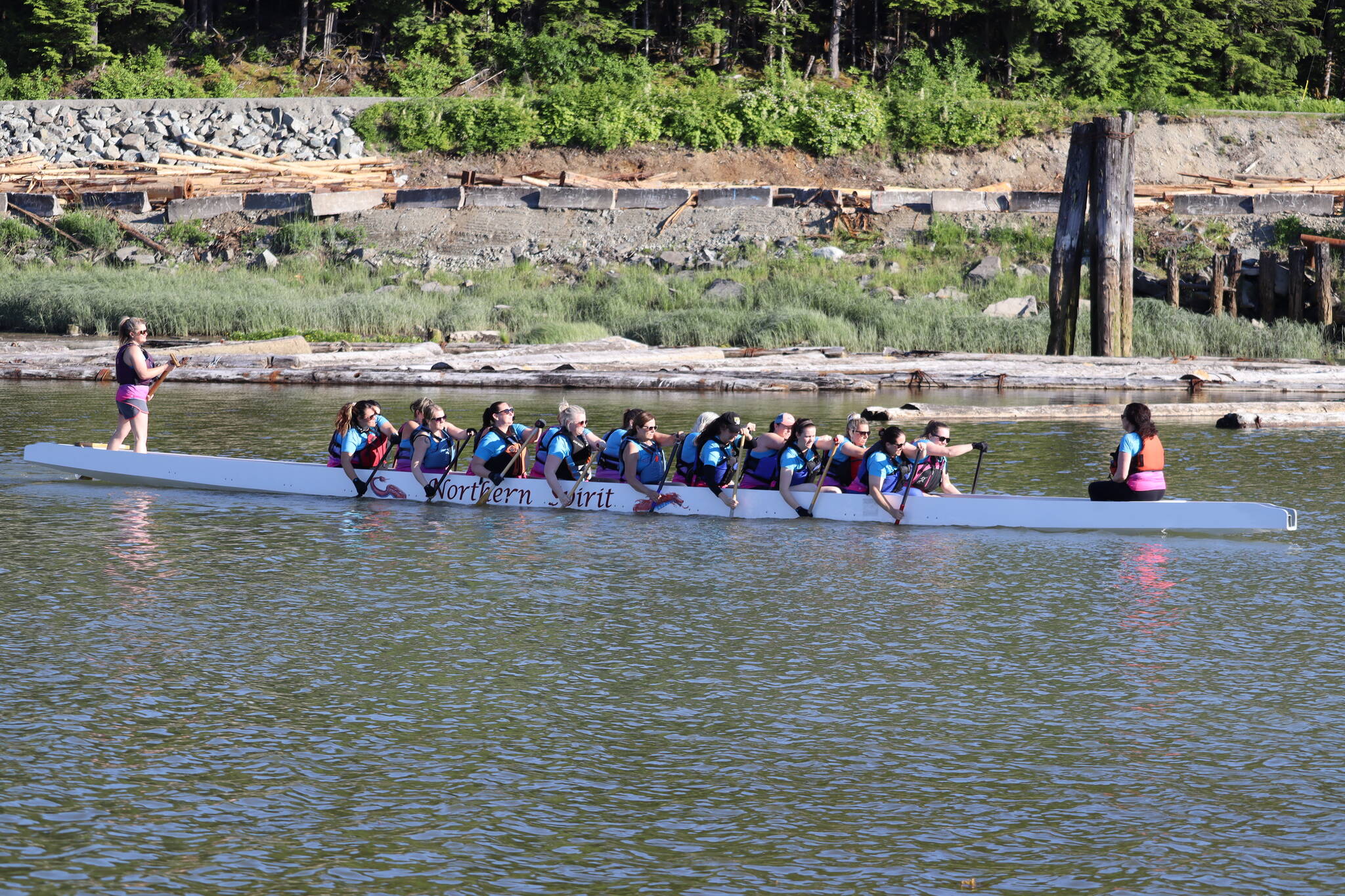This photograph captures a vibrant outdoor scene featuring a group of rowers preparing to navigate a long, white boat labeled "Northern Spirit" in a green waterway. The boat, resembling an elongated canoe, seats about 14 to 16 people arranged in pairs. Most of the rowers are wearing short-sleeved blue t-shirts and life jackets. At the front of the boat, a woman is seated in a red life vest, blue and pink shirt, and black leggings, while at the back, another woman stands in a black life vest, pink shirt, and gray shorts, holding a handle that likely controls the rudder. Surrounding the waterway, the backdrop includes a line of trees, a gravel road, and a pile of rocks adjacent to bushes. Construction barriers and more piles of dirt and wood are also visible, leading up to a cliff edge on the right. Logs tied together float close to the boat, and large, tall grass grows near the water's edge, adding to the natural setting. The atmosphere hints at a casual, enjoyable outing rather than a competitive race, suggesting that the rowers might be at a summer camp.